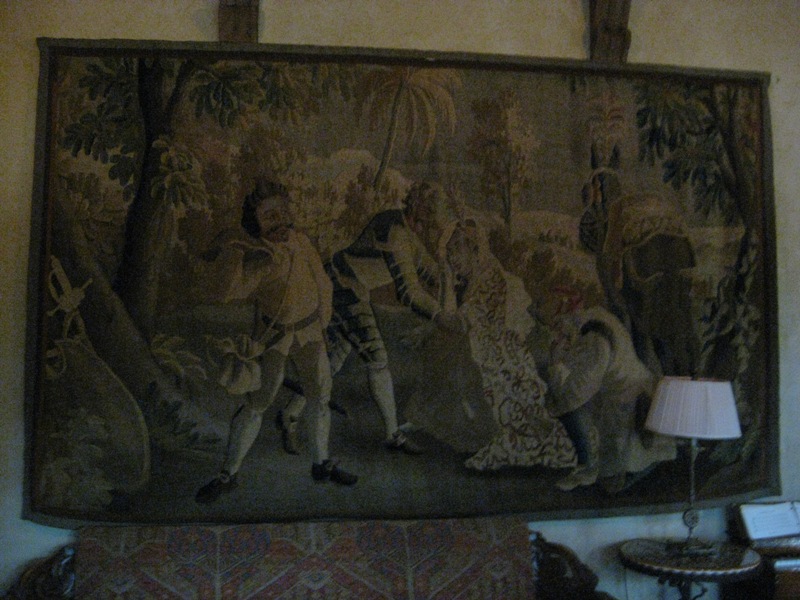The image showcases a large tapestry hanging on a white wall, which has tan markings and is dimly illuminated. The tapestry, rendered in muted tones of black, green, and gray, depicts a scene with tropical palm trees and lush greenery in the background. In the foreground, there are six people dressed in ancient attire. One man kneels beside an elderly woman, who appears to be in need of assistance, while another man stands to the left with a bag over his shoulder. On the right, there is an animal, possibly a horse or donkey, and several of the individuals seem to be interacting or conversing with each other. Below the tapestry, an elaborate scene unfolds with a small, elegant round table topped with a white lamp and a delicately crafted sofa. The room exudes a sense of historical ambiance and subdued elegance.